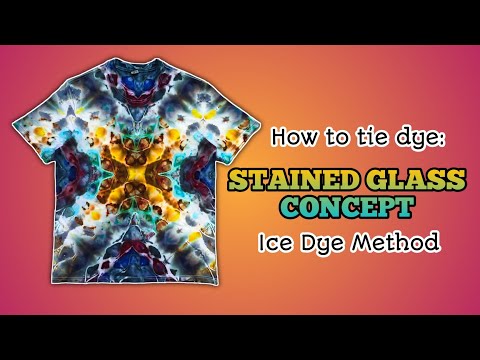The image is a webpage showcasing a tie-dye tutorial. On the left side of the image, there's a short-sleeved t-shirt with a tie-dye pattern that resembles an X shape, featuring vibrant colors such as yellow in the center, transitioning to brown, white, dark blue, greens, and purples. The t-shirt displays a kaleidoscope or stained-glass effect, achieved using the ice dye method.

On the right side of the image, there is text organized into several lines. At the top, prominent black letters outlined in white read "How to Tie-Dye." Below this, large yellow block letters with a slight light green gradient from the bottom spell out "Stained Glass." The next line features the word "Concept" in black letters bordered in white, transitioning from light blue at the top to blue at the bottom. Lastly, the line "Ice Dye Method" appears in the same style as the topmost text, with black letters surrounded by white. The background of the entire image is a gradient transitioning from red to orange, with black borders on both the top and bottom edges.